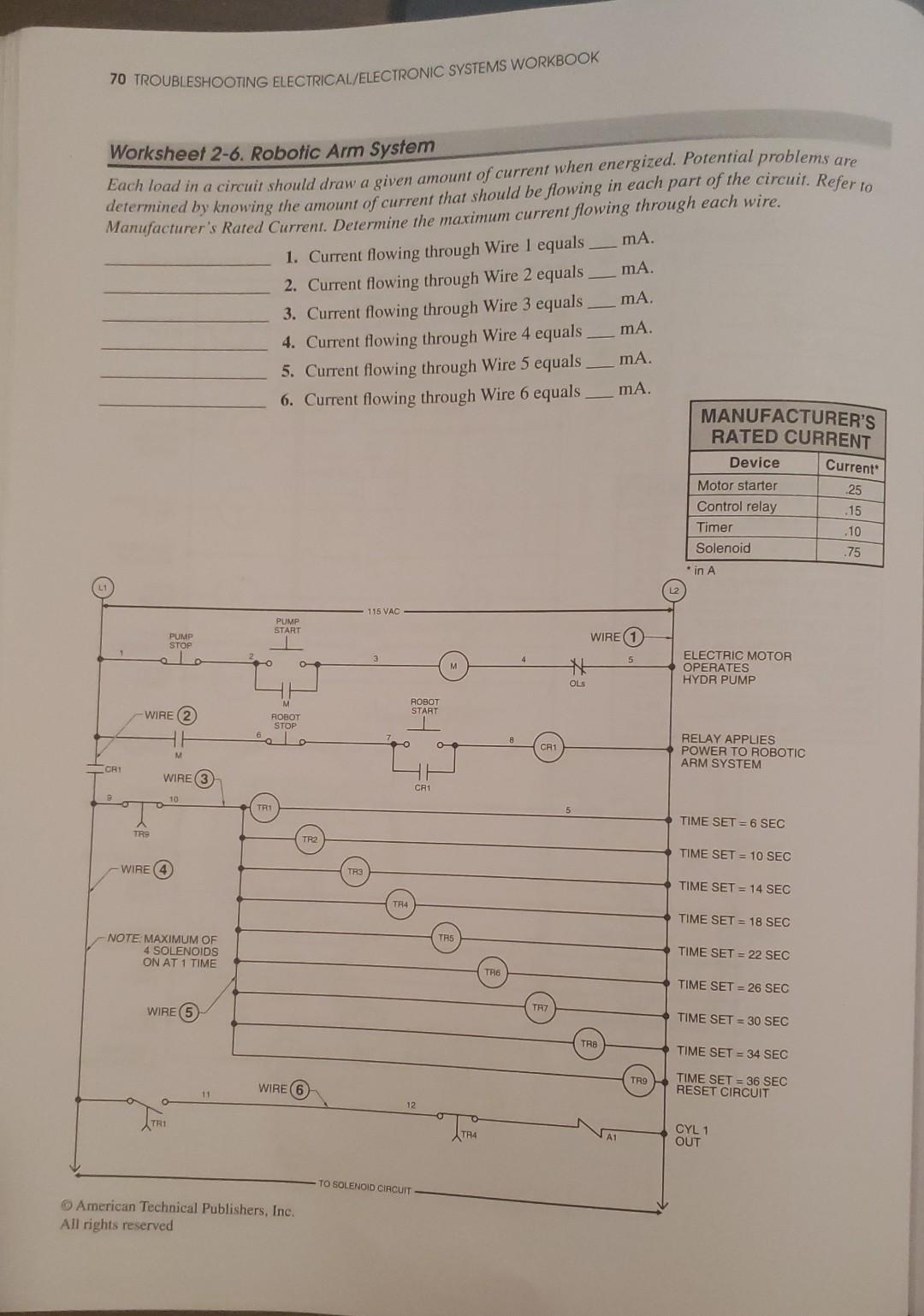This image captures a page from a workbook titled "Troubleshooting Electrical and Electronic System Workbook." It is on page 70 and features Worksheet 2-6, labeled "Robotic Arm System." The page is filled with various instructive elements and technical details. At the top, the title is prominently displayed, leading into detailed instructions about assessing potential problems by considering the manufacturer’s rated current for each device in the system. Central to the page is a list of four devices, each with its corresponding current rating: Motor Starter (0.25), Control Relay (0.15), Timer (0.10), and Solenoid (0.75). The worksheet appears interactive, containing numbered items intended to be matched with their corresponding answers. Toward the bottom of the page, an intricate diagram illustrates an electrical circuit, annotated with time settings ranging from 6 to 36 seconds and complex interconnections. Additional text along the side notes, "Electric Modem Operates Hydrant Pump," and a note at the bottom states, "American Technical Publisher, Inc., All Rights Reserved."